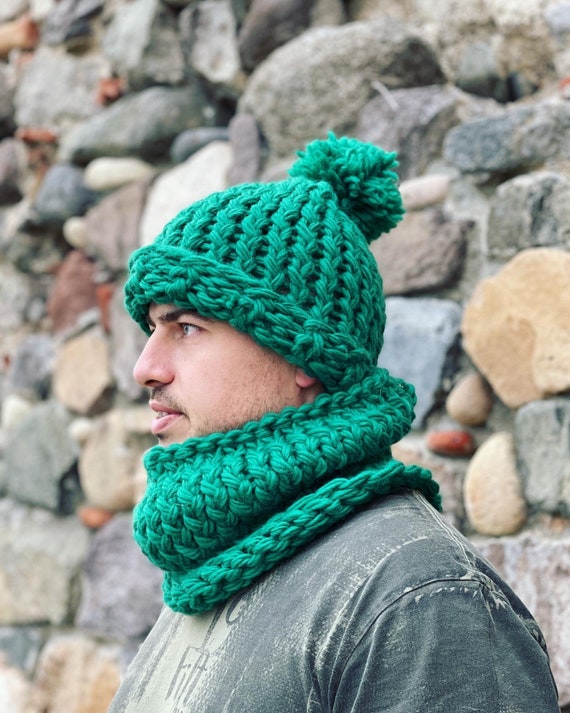In this photograph, we see a man with a lighter skin tone turned to the left, offering a clear side view of his upper torso and face. He sports a chunky-knit, bright turquoise-green beanie adorned with a large pom-pom, and a matching scarf. His facial features include dark eyebrows, a stubbly mustache, and partial beard growth, with his mouth slightly open and his ears covered by the beanie. He is dressed in a gray jean jacket over a textured, metallic blue shirt, possibly with some markings on it. The backdrop is a cobblestone wall composed of various sized and colored stones, ranging from earthy grays and browns to more vivid hues like light blue, orange, and maroon. Some stones are blurred, emphasizing the focus on the man.